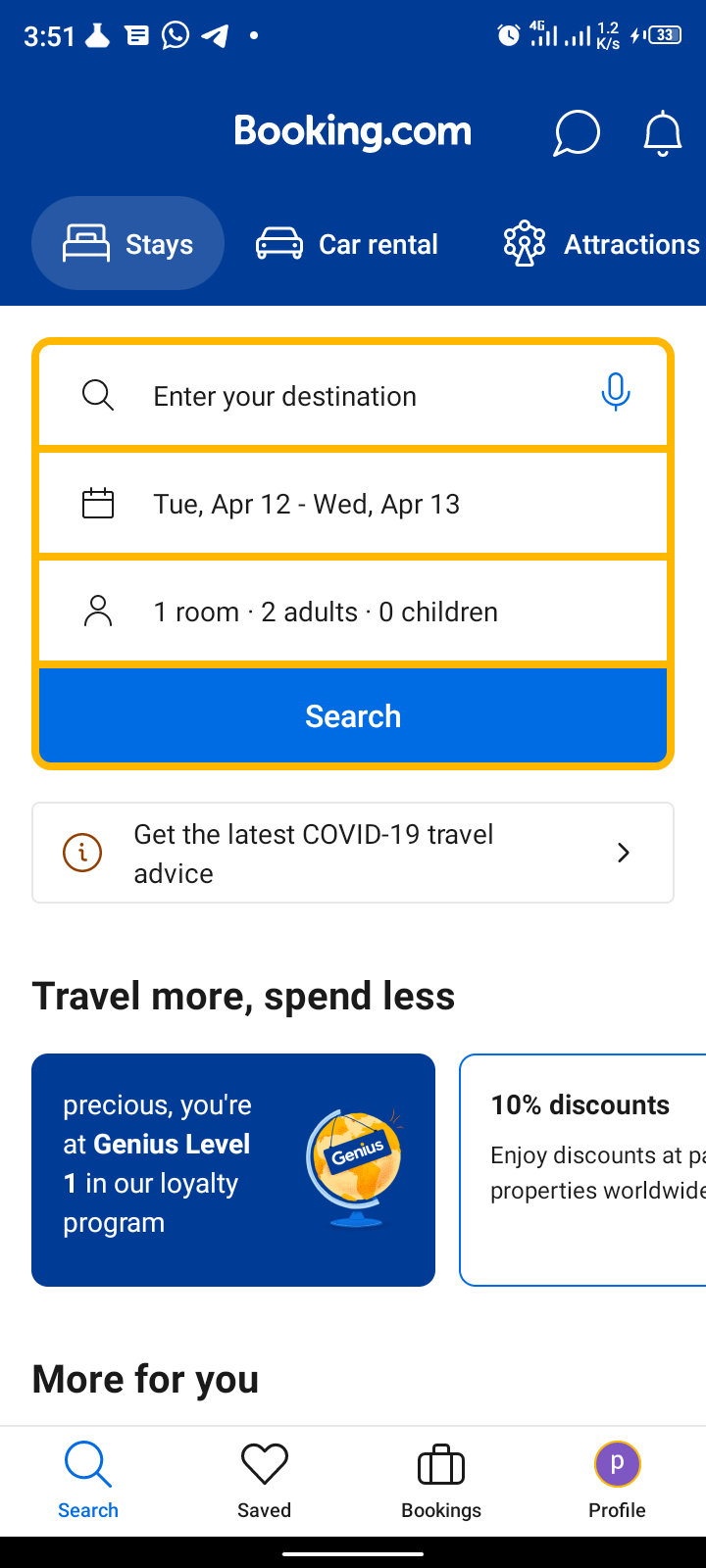A user is navigating the Booking.com app on their smartphone. The screen displays several sections for booking various services such as stays, car rentals, and attractions. The 'Stays' section is currently active, prompting the user to enter details like destination, check-in and check-out dates, the number of rooms, adults, and children. Below this form, a COVID-19 advisory section is visible, offering the latest travel advice with a clickable button for more information.

Further down, a promotional message appears, encouraging users to "Travel more, spend less." It acknowledges a user named "Precious" at a 'Genius Level 1' tier in the loyalty program, offering a 10% discount. The app's footer includes navigation options such as Home, Search, Saved, Bookings, and Profile, with the background predominantly white, accented by blue elements of varying shades.

The screen also shows a blue search button activated after inputting travel details. The notification bar includes some unique icons, including a lab beaker and various message-related symbols, adding an intriguing touch to the familiar interface.